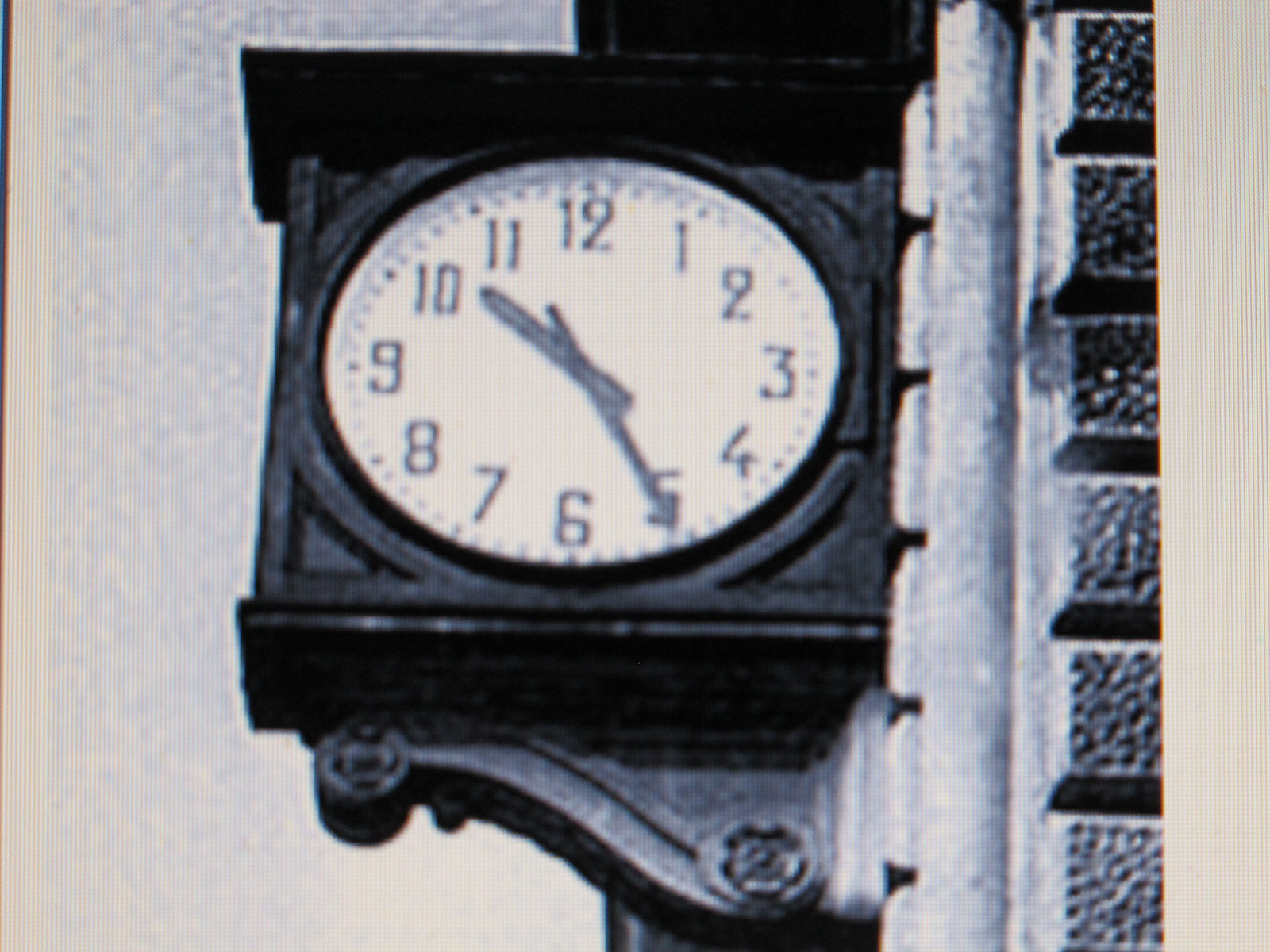A striking black and white photograph captures the side of a vintage brick building adorned with an elegant clock. The clock, mounted on the wall, features a classic design with a bold black outer rim and a standard analog face. The face displays numerals from 1 to 12 in a clockwise sequence, marked by dots that indicate the minutes. The minute hand, the longer of the two hands, points precisely at the 5, while the shorter hour hand hovers between the 10 and the 11, indicating a time of approximately 10:25. The monochrome tones emphasize the timeless quality of the scene, evoking a sense of nostalgia.